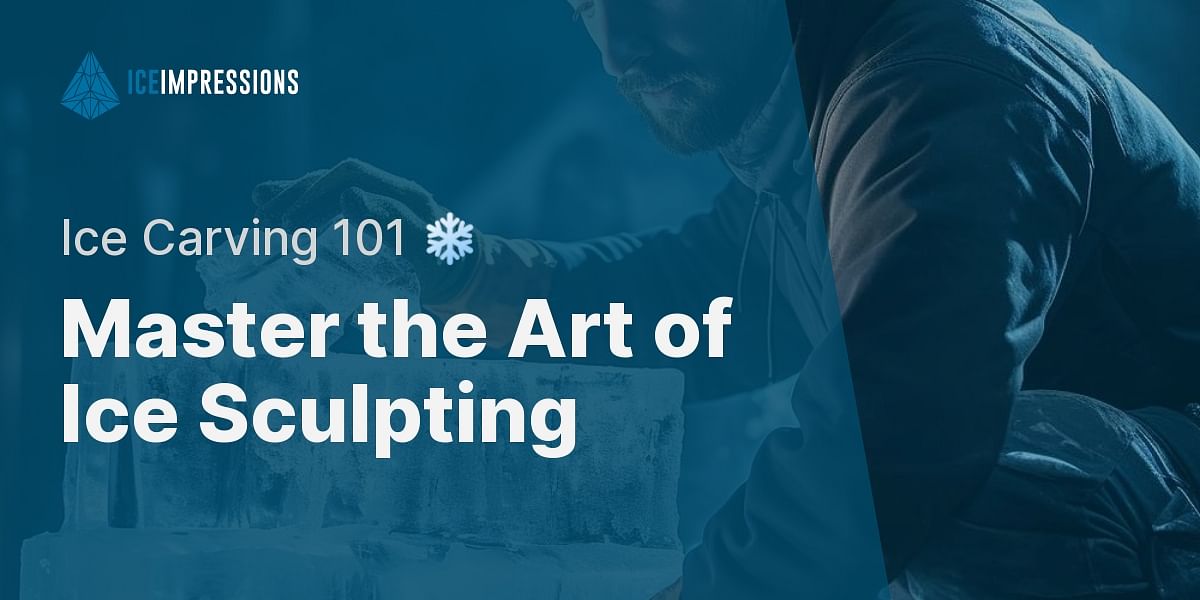The image depicts a billboard or poster with an oblong, rectangular shape, dominated by dark blues and black backgrounds. The central feature is a blue graphic with white text that reads "Ice Carving 101" alongside a white snowflake, and "Master the Art of Ice Sculpting" in bold, prominent letters. On the right side of the image, a bearded man dressed in warm clothing and wearing gloves is engaged in carving a block of ice. A unique diamond shape, possibly a logo reading "Ice Impressions," is also present near the top of the poster. The entire scene appears to have a blue tint, enhancing the cold, icy ambiance, and the background and parts of the man and the text have a frosty, film-like overlay, making it look like they are encased in ice.